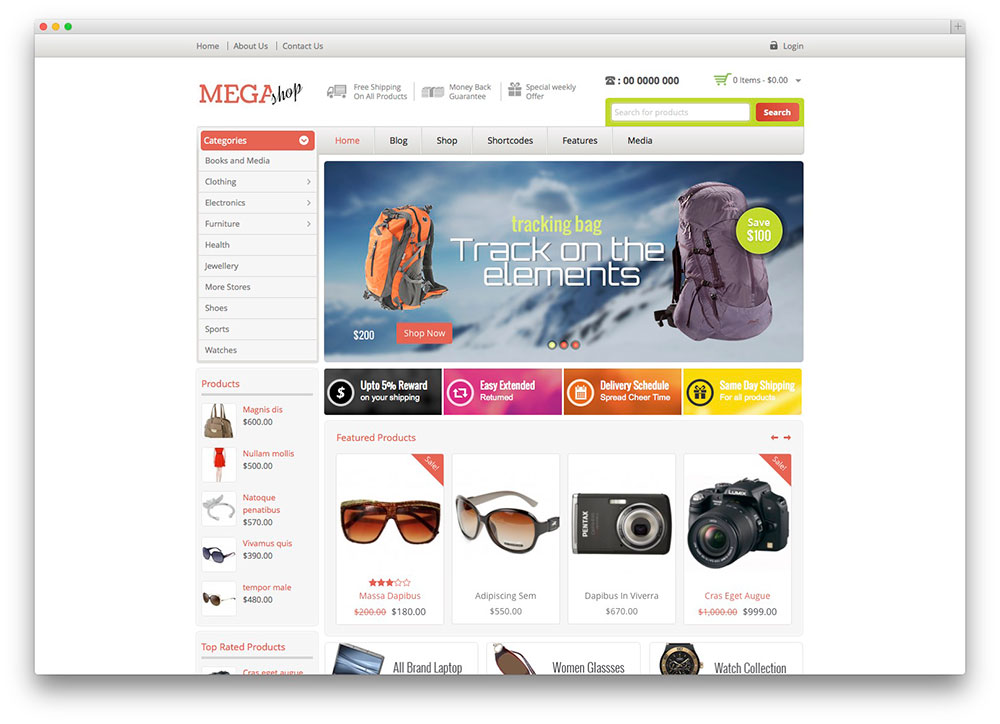This screenshot showcases a desktop view of an Apple device, displaying a website interface. The browser window design remains unidentified, lacking a visible web address bar. The image captures the website named "Mega Shop," prominently featured with "Mega" in red and "Shop" in black, using distinct fonts. The window's top-left corner includes standard Apple window controls—a red, yellow, and green circle, reminiscent of a horizontal traffic light.

The website's header contains navigation links, including "Home," "About Us," and "Contact Us," located on the left, with a "Log In" link to the right. Below this, visual icons depict services: a truck symbolizing "Free Shipping on All Products," a bundle of cash indicating a "Money Back Guarantee," and a gift box representing a "Special Weekly Offer." 

The absence of a legitimate contact phone number, represented by a series of zeros, suggests that this site is in a development or demo phase. The shopping cart icon indicates no items present. Users can search for products via an available search bar, reinforced by a secondary menu displaying options such as "Home," "Blog," "Shop," "Shortcodes," "Features," and "Media."

To the left, a vertical sidebar menu highlights product categories with a distinct design: a red rectangle with white text labels "Categories," followed by options like "Books and Media," "Clothing," "Electronics," "Furniture," "Health," "Jewelry," "More Stores," "Shoes," "Sports," and "Watches," each within white rectangles with black text. Expandable subcategories are noted for several entries.

Centrally, product thumbnails showcase various items with associated prices, interspersed with placeholder "Lorem Ipsum" text, clearly meant for demonstration purposes. On the right side of the screen, an advertisement features a hiking backpack labeled "Tracking Bag, Track on the Elements" priced at $200 with a promotional "$100 Savings" and a "Shop Now" call to action.

Further promotional banners, presented in black, pink, orange, and yellow rectangles with white text, advertise services such as "Up to $5 Reward on Your Shipping," "Easy Extended Returns," "Reschedule to Spread Cheer," and "Same Day Shipping for All Products."

Finally, the bottom section displays a range of featured products, including sunglasses and cameras. Additional categories like "All Brand Laptops," "Women's Glasses," and "Watch Collection" are previewed below, reinforcing the site's functionality as an online retail platform not yet finalized for public use.